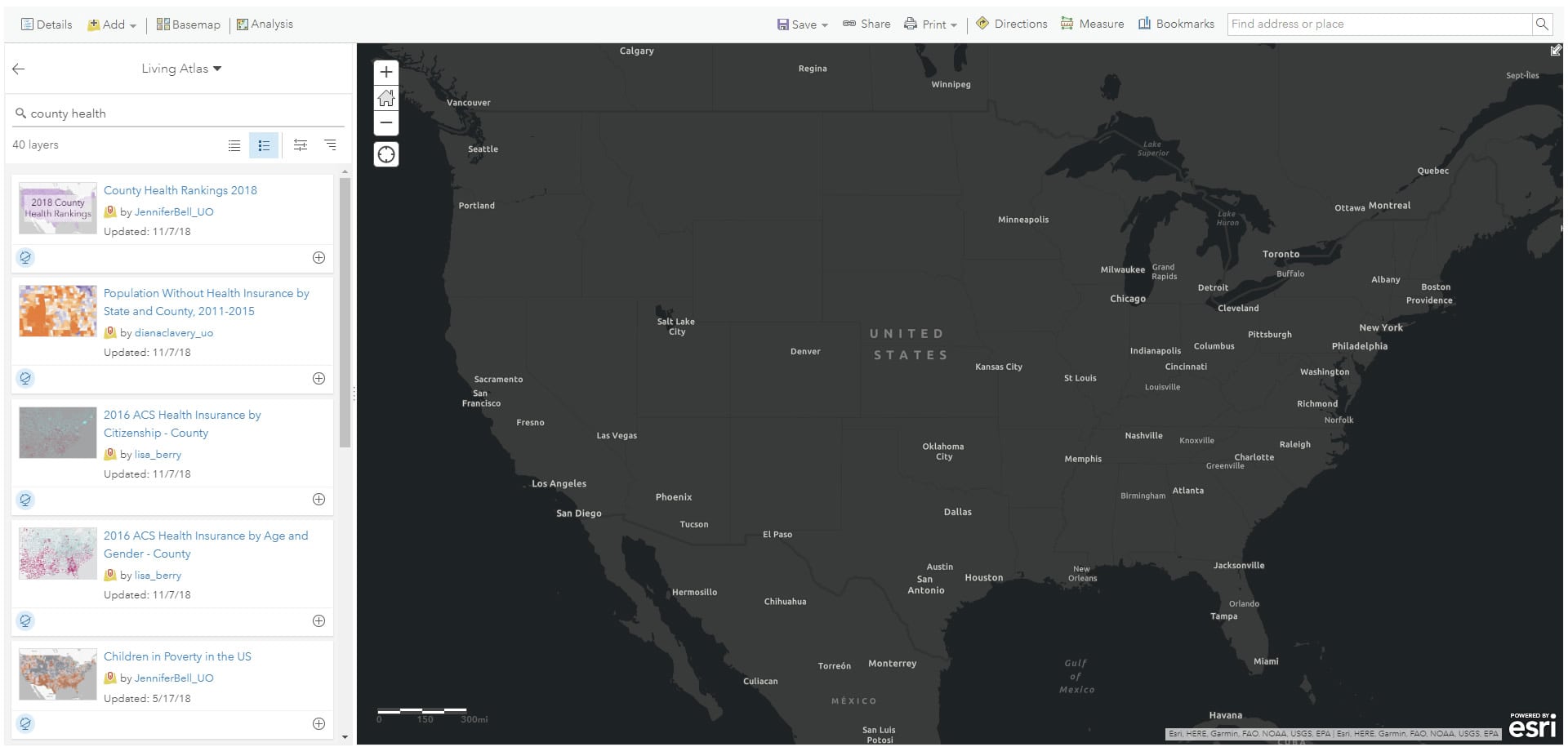To the right, there is a detailed map of the United States, extending slightly into Canada. The land areas are depicted in a neutral grey, while bodies of water are rendered in a darker grey. Prominent cities within both the United States and Canada are labeled in white for clear visibility. 

On the left side of the image, there is a vertical column consisting primarily of an advertisement and navigational options. At the top of this column, there are several clickable tabs labeled "Details," "Add," "Base Map," and "Analysis," which are likely related to the map's functionalities.

Below these tabs, a search query reads "county health," and a list of relevant links follows. These links include:

1. "County Health Rankings 2018"
2. "Population Without Health Insurance by State and County"
3. "2016 ACS Health Insurance by Citizenship by County"
4. "2016 ACS Health Insurance by Age and Gender by County"
5. "Children in Poverty in the U.S."

All these data points and resources were last updated in 2018, providing a comprehensive overview of various health statistics relevant to the United States.